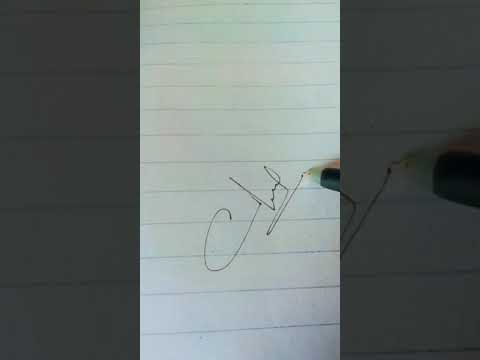The image showcases a person inscribing a somewhat illegible, cursive scrawl diagonally across lined paper. The inscription, starting with a capital 'C' or 'J', evolves into a series of intricate loops and flourishes, suggesting it might be a signature. The writing tool appears to be a pen, identifiable by its green-tipped point and darker green body. The image complexity is heightened by a zoomed-in, dimmer background that reveals a blown-up portion of the same paper, slightly darkened, adding depth and emphasis to the scene. This photograph captures the act of writing with a fine-tipped pen or possibly a pencil, against the backdrop of unevenly spaced lines due to the perspective of the shot.